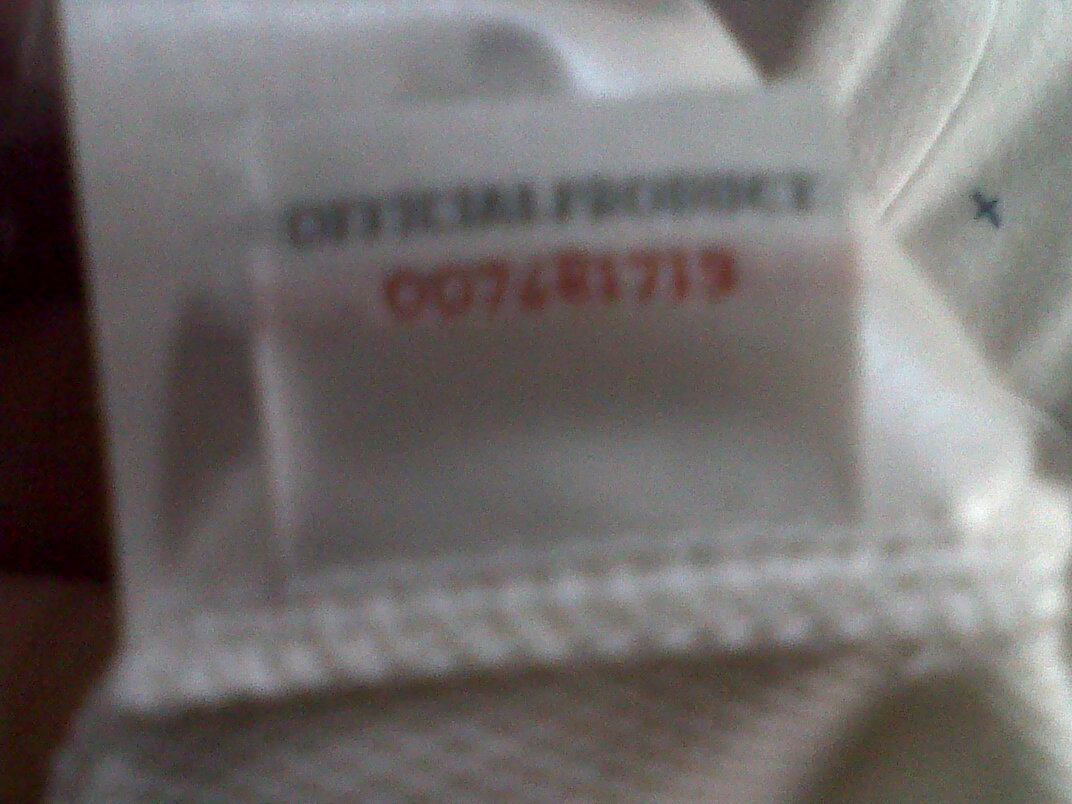The image is a close-up, landscape-oriented photograph of a white shirt's tag. The photo is extremely blurry and grainy, making details hard to discern. The white shirt and tag feature white stitching and a smooth tag material, contrasting with the more textured fabric of the shirt. The tag, which stands out in the upper left corner of the picture, bears the phrase "official product" in black lettering. Below this text, red numbers are visible, possibly reading 007481713, though the blurriness makes the exact sequence uncertain. In the background, there is additional white fabric, and a black X or cross mark is visible, enhancing the complex visual texture of the image.